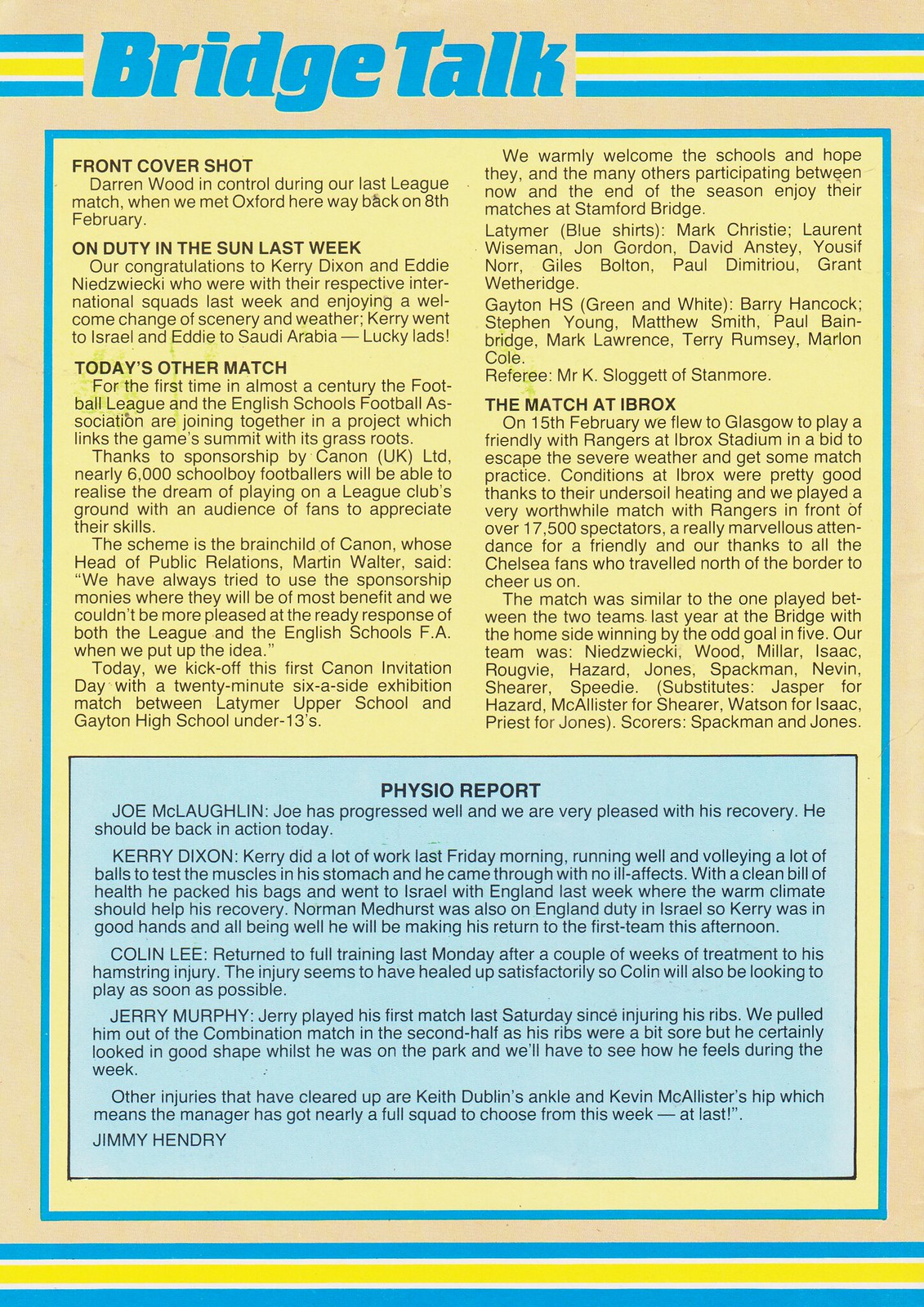The image depicts a large informational poster that occupies the entire frame, featuring a plethora of densely packed text and detailed updates related to football. The background of the poster is a cream color, bordered at the top and bottom by blue lines, with a central dividing line in yellow. At the top in bold blue font, the prominent heading reads "Bridge Talk."

The content is divided into several sections enclosed in a blue-bordered box. The first heading is "Front Cover Shot," mentioning Darren Wood in control during a league match against Oxford on February 8th. This is followed by "On Duty in the Sun Last Week," congratulating Kerry Dixon and Eddie Niedzwiecki for their involvement with international squads, with Kerry traveling to Israel and Eddie to Saudi Arabia. 

The middle section, under "Today's Other Match," discusses the unprecedented collaboration between the Football League and the English Schools Football Association, sponsored by Canon UK Limited. This initiative allows nearly 6,000 schoolboy footballers to play on league club grounds. The first Canon invitation day features a six-a-side match between Latimer Upper School and Gaten High School. Details of the teams, including names and jersey colors, are also included.

Another heading, "The Match at Ibrox," details a friendly game played on February 15th between Chelsea and Rangers at Ibrox Stadium, with a notable attendance of over 17,500 spectators. The Chelsea team lineup and substitutes are listed, along with the match outcome and scorers.

Below, in a prominent blue box titled "Physio Report," updates are provided on various players' recovery statuses. Joe McLaughlin's progress is highlighted, with him expected to return soon, alongside Kerry Dixon's successful recovery and participation with the English squad in Israel. Updates on other players like Collin Lee, Jerry Murphy, Keith Dublin, and Kevin McAllister are also detailed, reflecting a nearly full squad availability for the upcoming match.

The overall layout and dense information resemble something one might find in a school newspaper or a detailed article in a magazine, meticulously covering football-related events and player health updates.